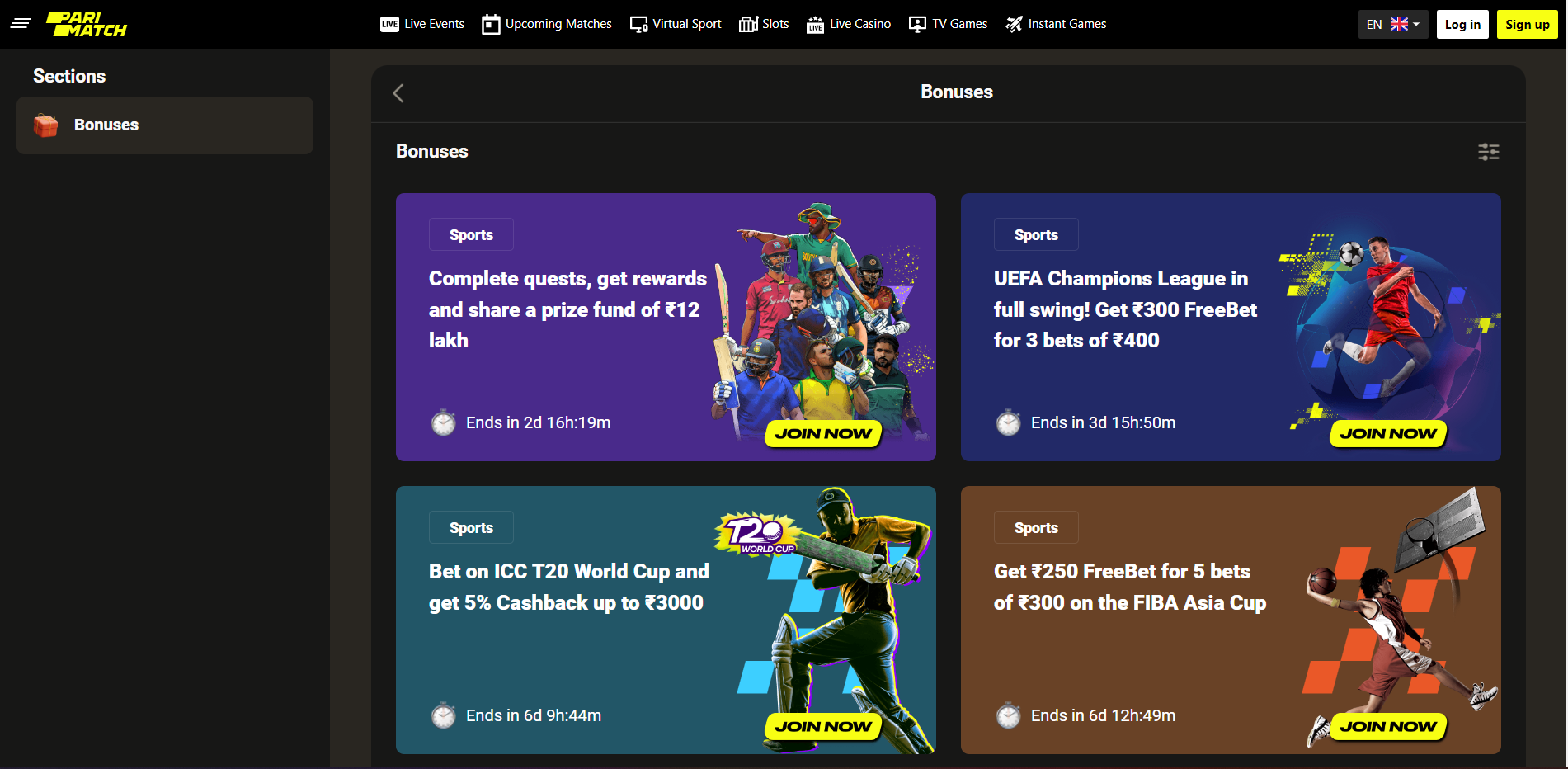This screenshot from a Parimatch interface captures various interactive elements and organized sections. At the top left corner, in yellow text, the title "Pari Match" is clearly visible. Aligned in the same row are multiple tabs labeled as Live Events, Upcoming Matches, Virtual Sport, Slots, Live Casino, TV Games, and Instant Games, providing easy navigation across different features.

The focal section displays the bonuses with four distinct colored boxes. The first box on the left is highlighted in purple and contains text detailing a sports-related quest: "Complete quests, get rewards, and share a prize fund of 12 EUR." The countdown timer indicates that this offer ends in 2 days, 16 hours, and 18 minutes. A "Join Now" button, prominently in yellow, invites user participation. The box is visually enhanced with computer-generated images of sports players including figures from cricket, soccer, and American football.

On the right side of the interface, the background transitions to blue, emphasizing UEFA Champions League activities with a tagline: "UEFA Championship League in full swing." Similar to the purple box, it includes a call-to-action "Join Now" button in yellow.

The remaining boxes also carry the theme of sports-related promotions, each containing a "Join Now" button in yellow ensuring uniformity and maintaining user engagement. The meticulous arrangements and visually appealing design elements provide a seamless and enticing user experience.